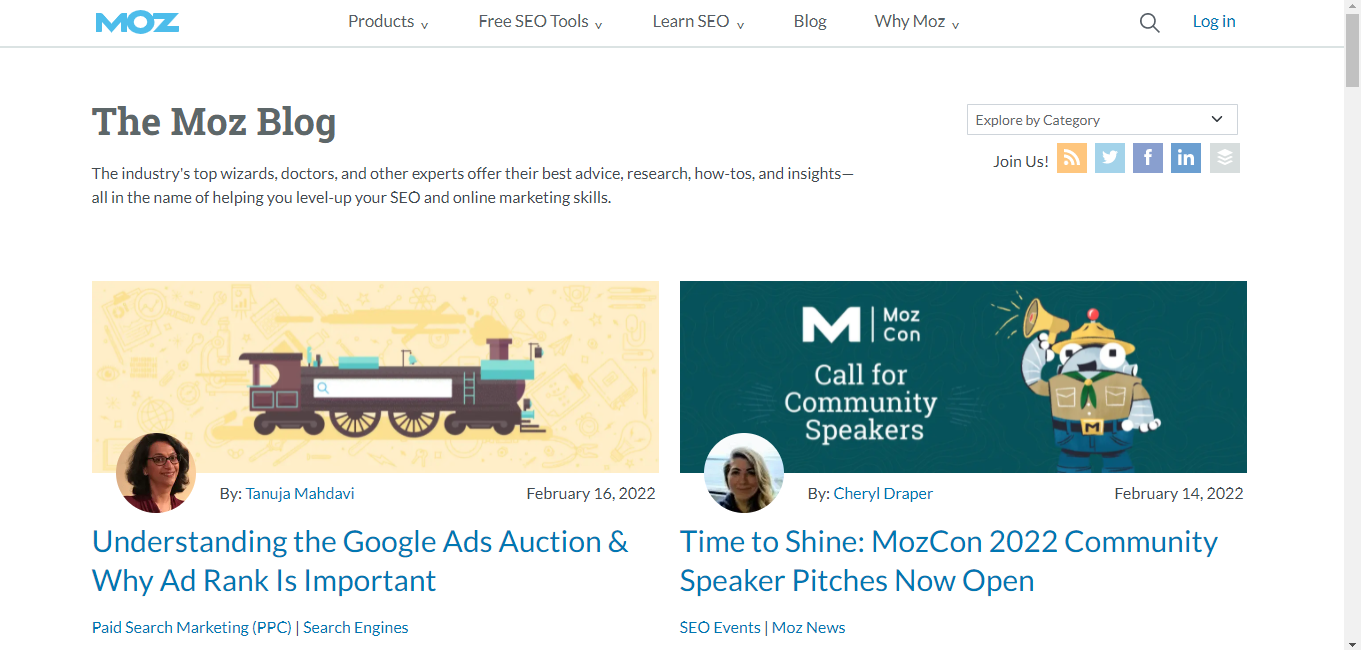The webpage displayed belongs to "The Moz Blog," a renowned platform in the SEO industry. At the top left of the page is the "MOZ" logo in blue, prominently placed in the header section. The main navigation bar includes tabs labeled 'Product,' 'Free SEO Tools,' 'Learn SEO,' 'Blog,' and 'Why Moz,' accompanied by a search icon and a 'Login' link in blue, while the rest of the tab labels are in black.

Immediately below the header, on the left side, is the title "The Moz Blog" followed by a descriptive text: "The industry's top wizards, doctors, and experts share their best advice, research, how-tos, and insights, all to help you level up your SEO and online marketing skills." Adjacent to this, on the right, is a dropdown menu titled "Explore by Category," allowing users to choose between different content categories. Beneath this menu, there are social media links labeled 'Join Us,' including icons for LinkedIn, Twitter, Facebook, and more.

The central section of the page, towards the right, features a highlighted announcement with white text on a dark green background: "MozCon Call for Community Speakers." Below this headline is an image of a cartoon character alongside a user profile. The profile belongs to Cherry Tripper, who posted on February 14, 2022, with the headline: "Time to Shine: MozCon 2022 Community Speaker Pitch is Now Open," categorized under 'SEO Event' and 'Moz News.' This text is written in blue.

To the left of this announcement is another blog entry featuring an image of a train set against a brown background. Authored by Tanuja Madhavi, the post has an illustrative profile picture and includes the headline: "Understanding the Google Ads Auction and Why Ad Rank is Important," categorized under 'Paid Search Marketing PPC' and 'Search Engines.' This descriptive text is also rendered in blue.